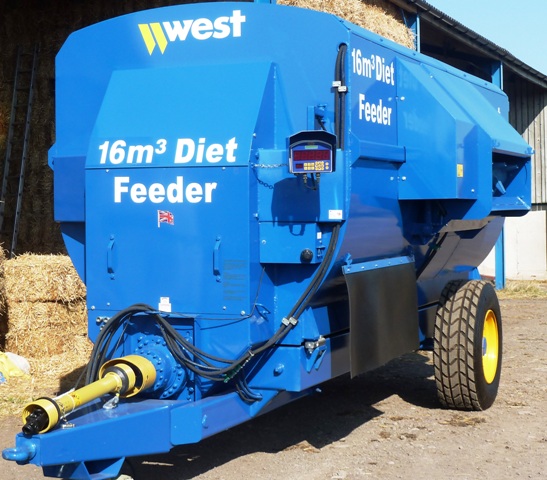The image showcases a detailed, diagonally positioned view of a large industrial machine, specifically a feeder. The prominent text on the machine reads "West 16 m³ Diet Feeder." The machine is a striking blue color with several recognizably distinct components, including black rubber tires with yellow centers. The front portion of the feeder features a long, tubular design and a hitch, suggesting it can be towed, though it appears unhitched in the image.

Positioned to the right of the machine, near its back, sits a visible wheel. Atop the feeder, there is some hay, indicating its agricultural use. The setting is an outdoor farm environment, with the machine resting on dirt and flanked by elements like a barn and a white building in the background. The photo was taken in daylight under a clear, bright blue sky. The colors visible in the image include various hues such as tan, brown, dark blue, yellow, white, black, and a touch of silver from the tubing and cables.